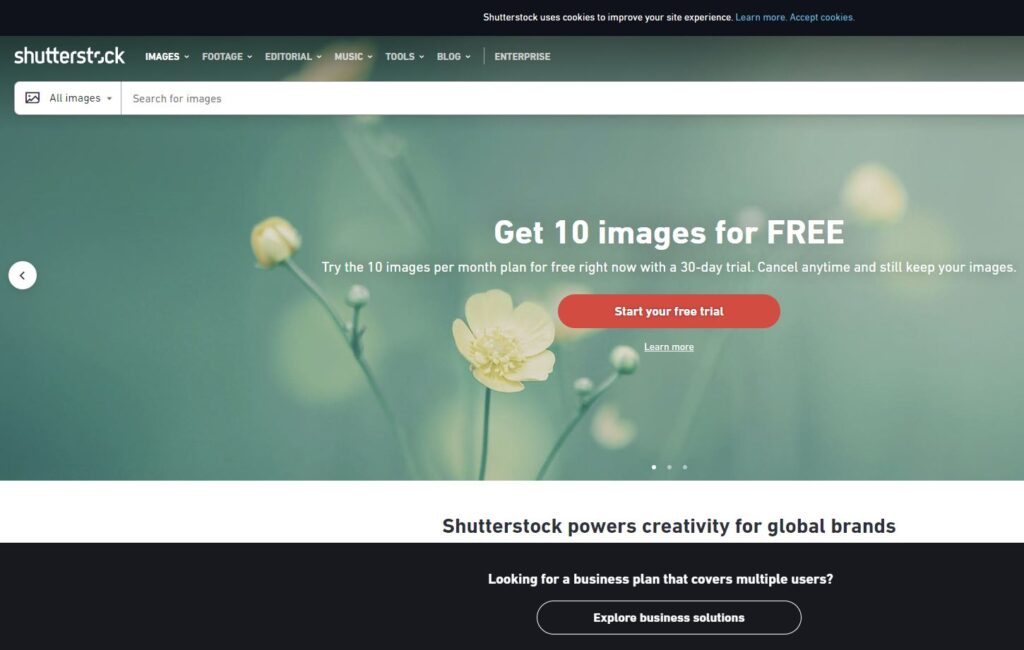The top portion of the image features a long, black rectangular bar with small white text that reads, "Shutterstock uses cookies to improve your experience." Directly beneath this bar, there is the word "Shutterstock" with a diagonal line running through the letter "O." To the right of "Shutterstock," there are several navigation options listed: "Images," "Footage," "Editorial," "Music," "Tools," "Blog," and "Enterprise."

Below this, there's a prominent long white search bar labeled "Search for images." The background of the main section of the image is green, adorned with a few beige or off-white circles. Emerging from the center are green stems, one of which has petals that are not fully opened, revealing they will be light yellow. Another stem in the center has fully blossomed, showcasing delicate, thin, light yellow petals.

In the upper part of the central section, white text encourages users to "Get 10 images for free." Beneath this, additional text elaborates: "Try the 10 images per month plan for free right now with a 30-day trial. Cancel anytime and still keep your images." At the bottom, there is a red circular button with white text that reads, "Start your free trial." Below this button, "Learn more" is underlined in white.